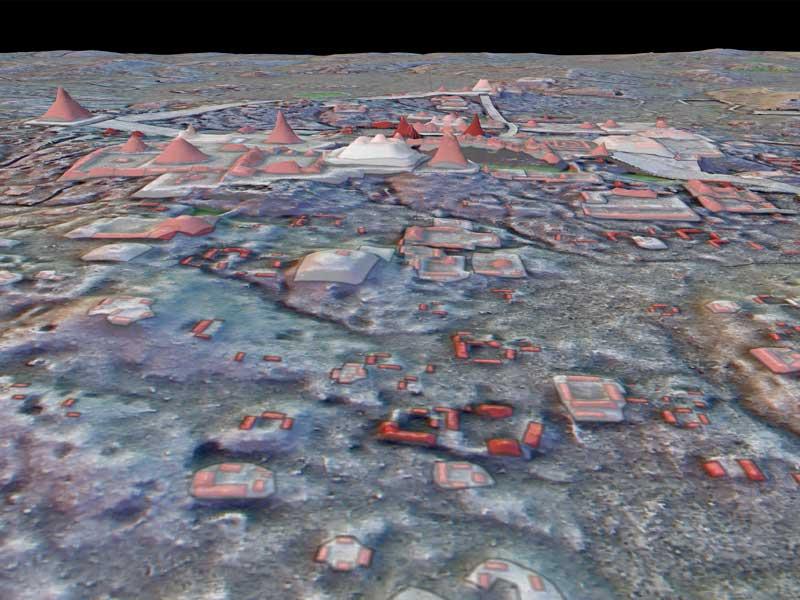This image is a detailed 3D rendering of a surreal, digital landscape viewed from a bird's eye perspective. It features a variety of geometric shapes and formations, predominantly pyramids, scattered across the scene. The bottom half of the image is relatively flat, while the middle to upper portions showcase an array of rising structures extending from left to right. The top eighth of the background is entirely black. The color palette includes shades of salmon, black, white, red, gray, blue, and subtle hints of purple. This landscape bears a resemblance to the LiDAR mappings used to uncover hidden Mayan temples and structures, with conical and pyramid-like shapes dotting the terrain, reminiscent of a city center and smaller village-like structures in the foreground. This composition may represent an alien or fantastical terrain, blending elements of a digital blueprint with the aesthetic of an ancient, possibly extraterrestrial, civilization.